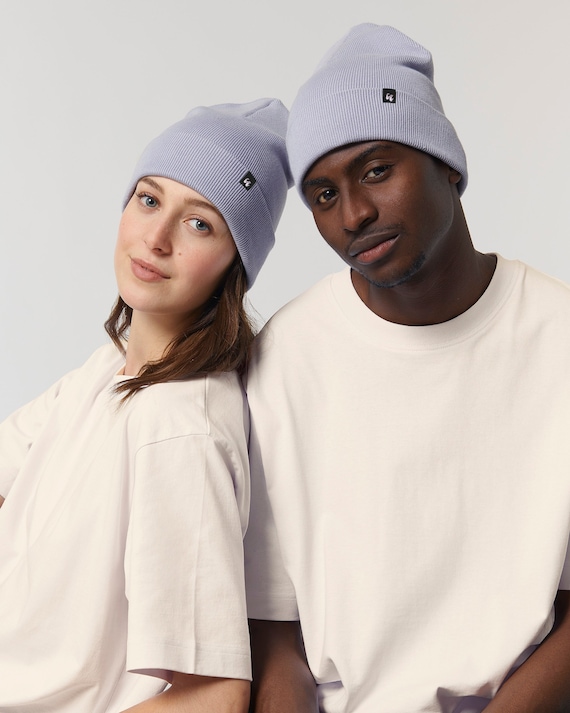This professionally posed, full-color photograph features two young models showcasing a unisex clothing line. The image, vertically rectangular with no visible border, is set against a plain light blue background that offers no distractions. The models are seated shoulder to shoulder, with the woman on the left leaning her back against the man's right shoulder. Both are looking directly at the camera, each sporting a slight closed-mouth grin.

They are dressed identically in short-sleeved white crewneck t-shirts and light blue beanies. The beanies are adorned with small black tags that feature what looks like white logos, possibly two C's or quotation marks, though the markings are too small to discern clearly. The woman has light-colored skin and blue eyes, with her shoulder-length brown hair cascading down to his shoulders. The man has dark skin and keeps his hair concealed under his beanie.

Visible parts of their arms and forearms add a casual touch to the otherwise minimalist composition, suggesting the photo is intended to highlight the versatility and appeal of the clothing items being modeled.